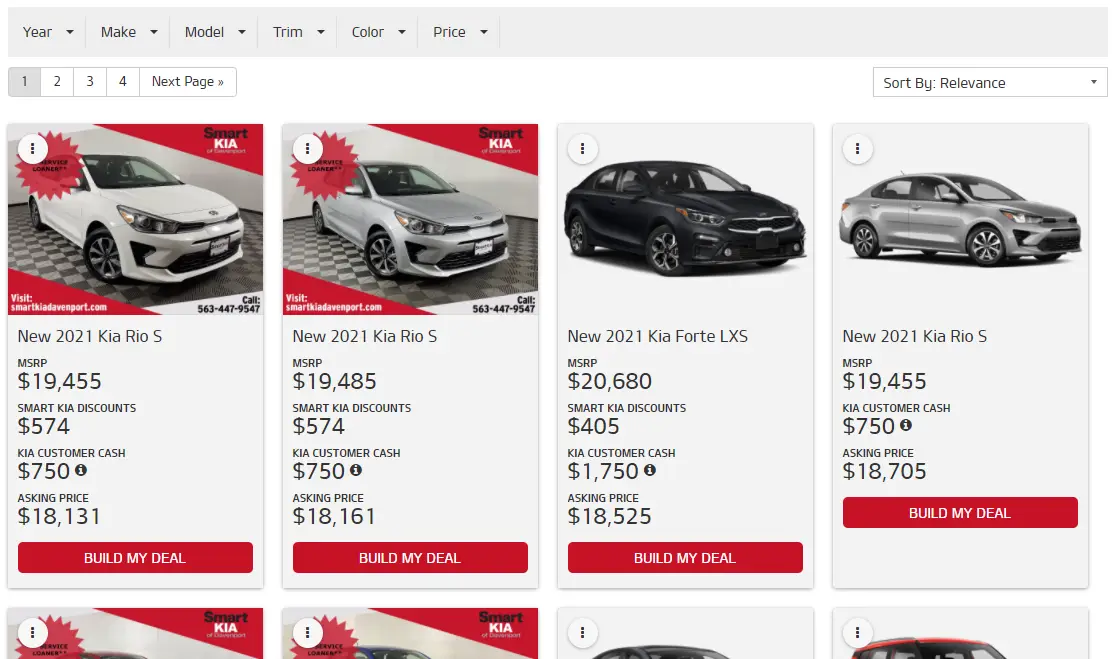This image features a detailed view of an online car dealership's webpage, specifically highlighting a selection of Kia vehicles. The top section of the page includes a navigation bar with filters for year, make, model, trim, color, and price. Below this, pagination options are visible, with page one highlighted in gray and options to navigate through pages one to four, including a "next page" button.

The main focus of the image showcases four vehicle listings. The first vehicle is a new 2021 Kia Rio S, priced with an MSRP of $19,455. After a Smart Kia discount of $574 and a Kia customer discount of $750, the asking price is $18,131. A prominent red "Build My Deal" button accompanies each listing.

Following is another 2021 Kia Rio S, priced at $19,485. After discounts of $574 from Kia and $750 in customer cash, the reduced price is $18,161, also accompanied by a "Build My Deal" button.

The third listing presents a 2021 Kia Forte LXS, with an MSRP of $20,680. After a $405 Kia discount and $1,750 in customer cash, the final price stands at $18,525, featuring the "Build My Deal" option as well.

Lastly, the image includes a 2021 Kia Rio S, initially priced at $19,455. Accounting for a $750 customer cash discount, the final price is $18,705.

Notably, the page includes a sorting option labeled "Sort by Relevance" and indicates that additional vehicle listings are available below the visible section. This webpage appears to be part of a car dealership's site dedicated to selling new Kia cars.